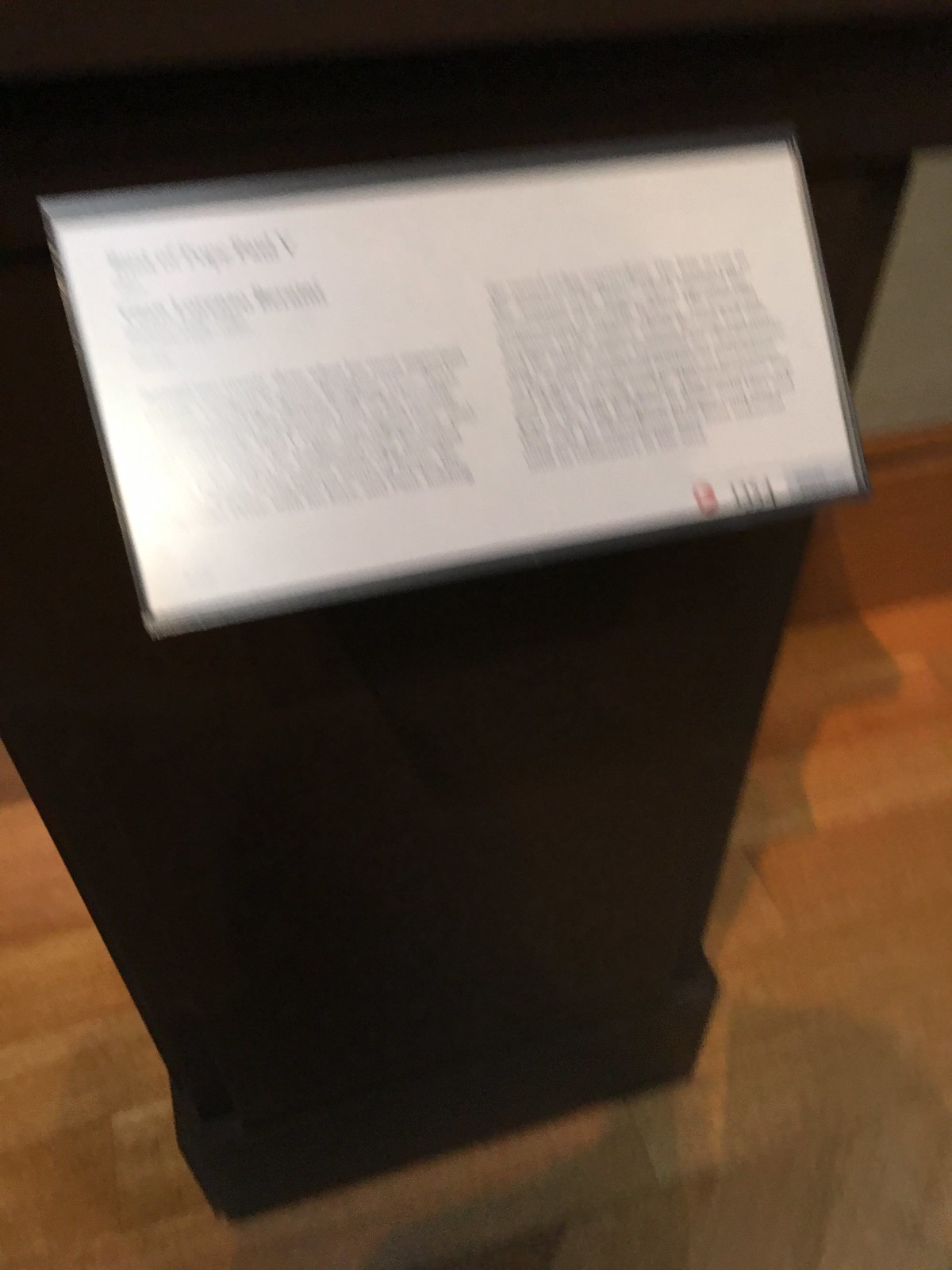A very blurry image features a sign situated on a tall, black rectangular pedestal, likely in a museum setting. The top of the pedestal is at eye level with the camera, casting a shadow over the white sign attached beneath it. The sign consists of a laminated piece of white paper with black text, including a title at the top followed by two paragraphs of writing—one on the left, slightly shorter than the one on the right. Unfortunately, due to the blurriness, the text is illegible. The floor is composed of wooden floorboards running horizontally across the scene.